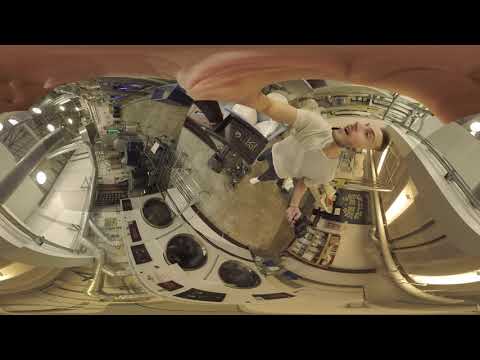The image captures a young man in a laundromat, taken with a fishbowl or fish eye lens, creating a distinctive panoramic effect with black borders at the top and bottom. The man, dressed in a white short-sleeve button-down shirt, dark pants, and white shoes, stands on a concrete floor that appears grayish-brown. Fluorescent tube lights and additional spotlights are installed in the ceiling above, which also features visible steel air ducts.

The man has dark hair, some stubble, and his mouth is slightly open, possibly talking, while he looks off to his left. His hand is prominently smeared across the top of the image, indicating motion, suggesting he used a selfie stick or inadvertently caught his hand in the frame while taking the photo. On the bottom left, a row of front-loading washing machines is visible, hinting at the laundromat setting. The walls are grey, and there seems to be clutter or storage behind him, possibly indicating that the laundromat is in a basement or an area with additional storage. Overall, the image depicts a typical laundromat scene with the added dynamic of the man's movement and the lens's distortion.